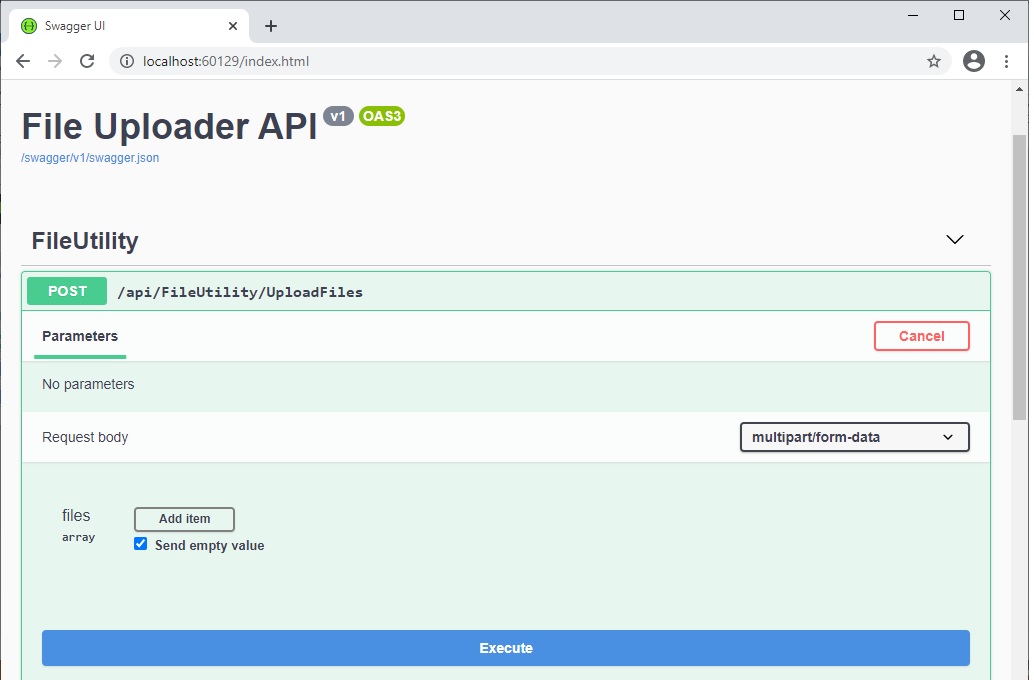Screenshot Description of Swagger UI Interface:

This image is a screenshot depicting the Swagger UI interface. At the very top, the browser address bar displays the URL: "localhost:60129/index.html". Below this, the API path is shown as "file loader API V1 OAS3/swagger/v1/swagger.json".

The main content area presents the Swagger UI for the "file utility" service, specifically the POST method available at the endpoint "/api/file utility/upload files". This endpoint does not require any parameters as indicated by the label "parameters: no parameters".

The "request body" section specifies the data type as "multi-part/form-data". Within this section, there is an option to upload files, represented as a "files array". Users have the ability to add additional items to the array using an "add item" button.

There is a checkbox located under the "send empty value" option, which is currently checked.

At the bottom of the interface, a prominent blue rectangle button centered horizontally contains the word "Execute" written in white letters.

The image is free from any photographic elements. It contains no people, animals, buildings, plants, flowers, trees, automobiles, motorcycles, bicycles, boats, airplanes, or helicopters.